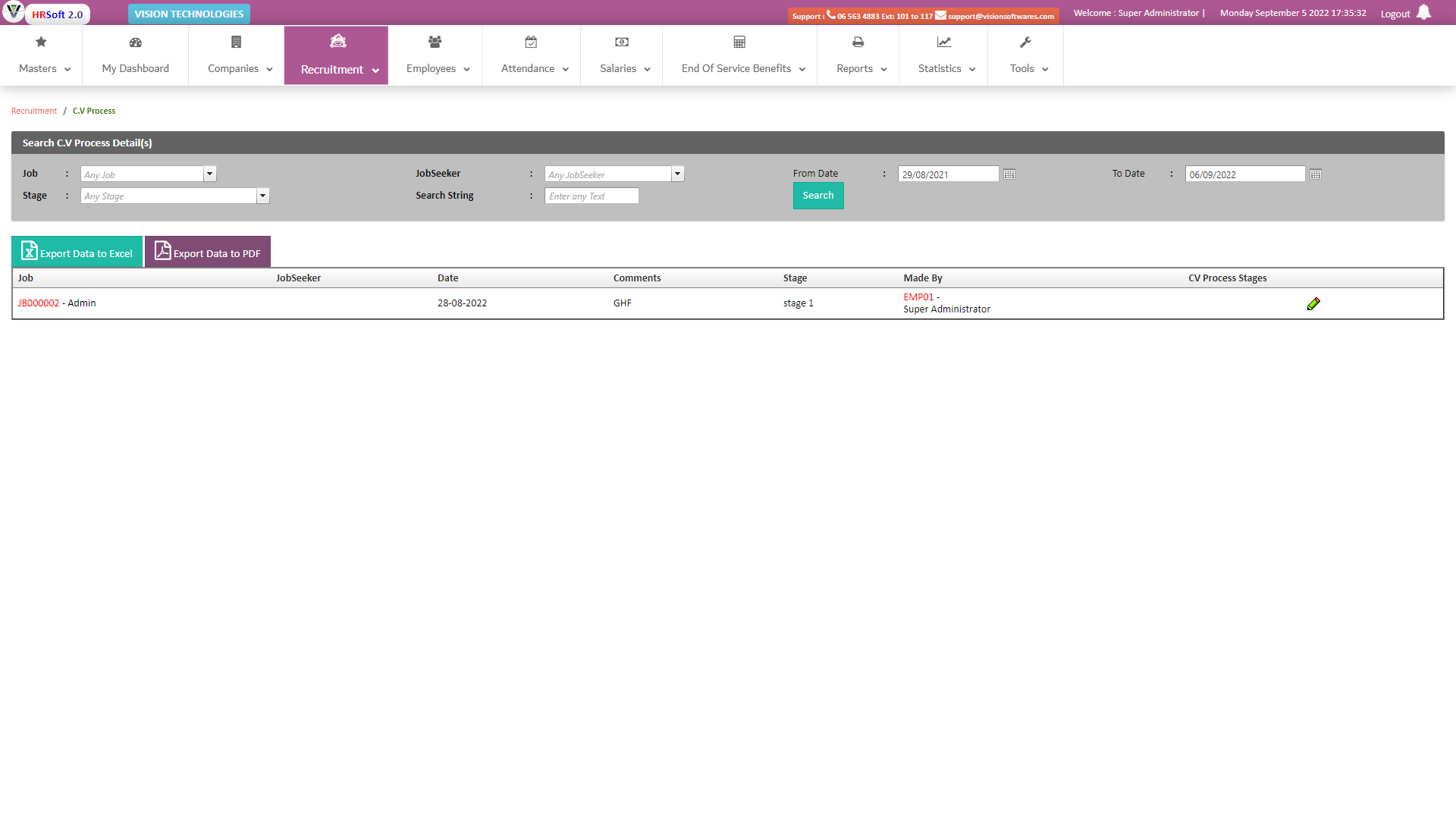The image displays a section of a web page designed for managing human resources. In the top left corner, there's a logo featuring a white circle that encompasses an inverted pyramid missing its top line, adjacent to the text "HR soft 2.0". The letters "HR" are in red, "soft" in blue, and "2.0" in a grayish tone, all set on a white, oval-shaped button. Next to this, in a green rectangle with white letters, is the title "Same Vision Technologies".

These elements occupy the topmost part of the page, followed by a navigation bar containing multiple tabs: "Masters", "My Dashboard", "Companies", "Recruitment", "Employees", "Attendance", "Salaries", "End-of-Service Benefits", "Reports", "Statistics", and "Tools". This indicates the web page is part of a comprehensive human resources management system.

Below the navigation bar, the current section is titled "Recruitment / CV Process". Underneath this title is a long, narrow gray box with six menu options, including fields for the job seeker's name, the job description, stage of recruitment, and other related details. At the bottom of this gray box, there are two action buttons: a green button labeled "Export Data to Excel" in white text, and a purplish button labeled "Export Data to PDF" in white text.

Further down, there's a list displaying job details, including a job number indicated in red next to the word "Admin". The list also includes columns for the date, comments, stage of recruitment, and other relevant information, emphasizing the functionalities related to managing recruitment processes within this human resources platform.